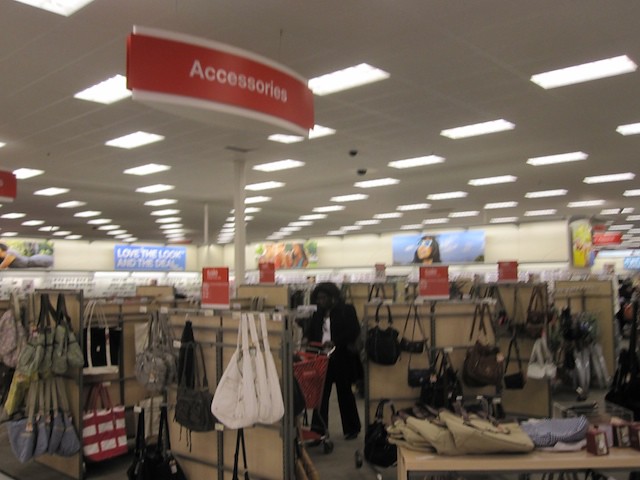This vivid color photograph captures the interior of a Target department store, specifically focusing on the bustling accessories section. The vantage point offers a bird's-eye view over a myriad of displays featuring various handbags and purses. Temporary walls are strategically positioned around the department, adorned with an array of stylish bags.

On the left side, one can see an assortment of beach-style bags, while the right side showcases larger, casual hobo bags. Further to the right, the selection transitions to more elegant, dressy handbags, catering to different tastes and occasions. Suspended above the displays, a prominent red sign spells out "Accessories," indicating the department.

In the background, a large blue sign mounted on the back wall encourages shoppers with the phrase "Love the Look and the Deal." Among the shoppers, a notable figure is a woman dressed in a sleek black pantsuit paired with a crisp white shirt. She navigates the accessory aisles with a red Target shopping cart, reinforcing the store's identity. Her black hair contrasts sharply with her outfit, making her stand out in the lively scene.